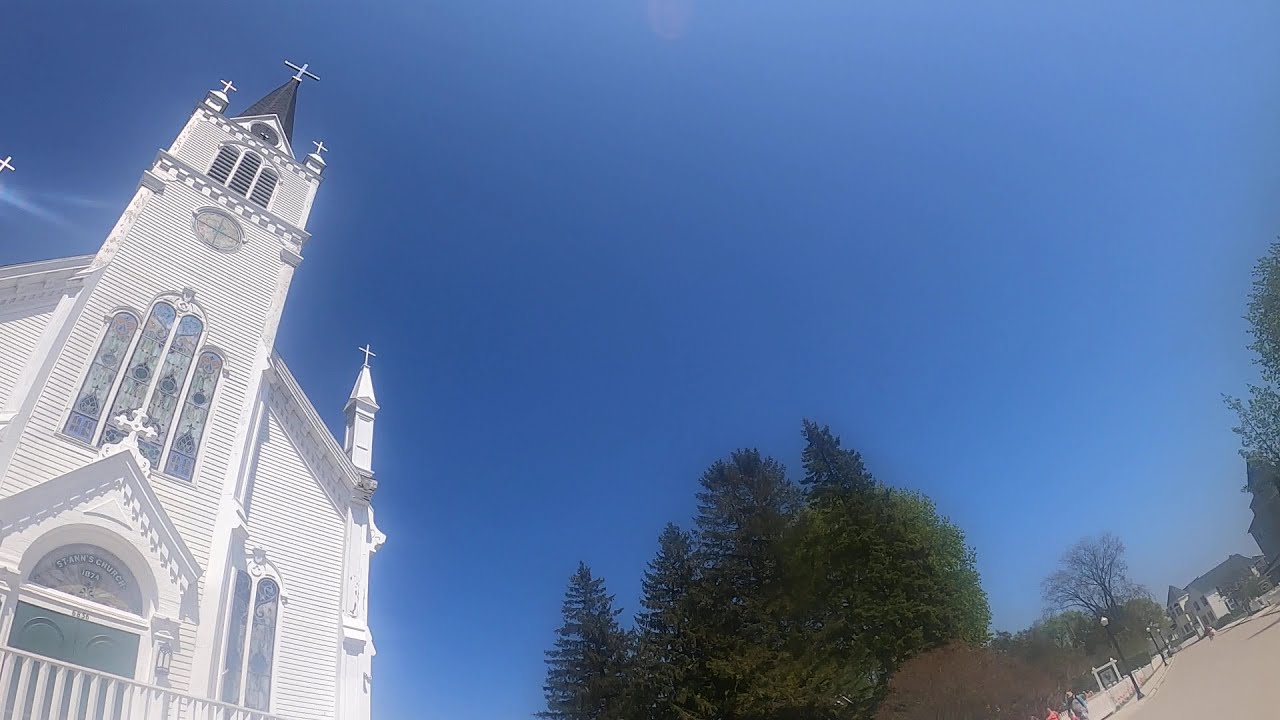In this captivating daytime photograph, taken close to the ground with an upwards angle, a prominent white church dominates the left side of the image. The church features a tall central spire topped with a cross and flanked by two smaller spires, each also crowned with crosses. Beneath the spires, the church showcases elegant tall stained glass windows, adding to its grandeur. At the base of the structure, a green door is set into an archway. To the right of the church, a cluster of large, green fir trees provides a natural backdrop. The sky overhead is a vibrant blue, almost entirely clear except for one wispy cloud on the left. On the bottom right corner of the scene, a street can be seen, leading towards a white house with a dark roof in the distance. The street and sidewalk are sparsely populated, with a few tiny figures visible, highlighting the spacious and almost tranquil setting of this sunlit day.